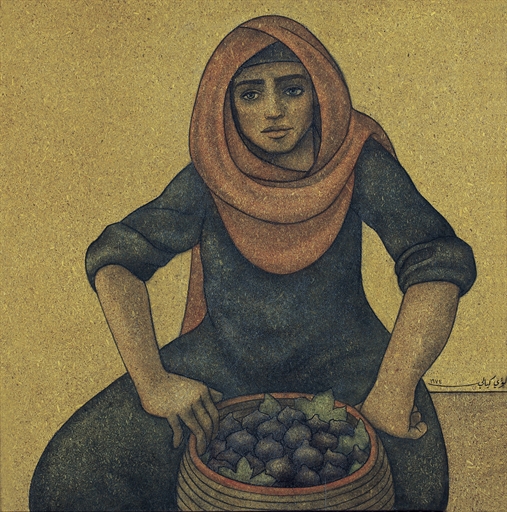The image features a hand-drawn or painted artwork of a woman sitting in the center against a tan to brown background. She is wearing a long, plain, dark blue gown with her sleeves rolled up to her elbows, and a pink headscarf covering her head. The scene has an old, timeless look to it. The woman, who appears to be situated in an old city setting, sits with her legs covered by the dress but with her knees apart. She has a woven basket, filled with dark purple fruit resembling black plums or figs, positioned between her legs. Details include green leaves emerging from the basket, and the woman’s hands rest on her legs as she gazes off into the distance. In the bottom right corner of the image, the artist's signature is visible. The overall color palette features shades of blue, pink, tan, brown, green, and a touch of off-red, lending a rich, textured feel to the scene.